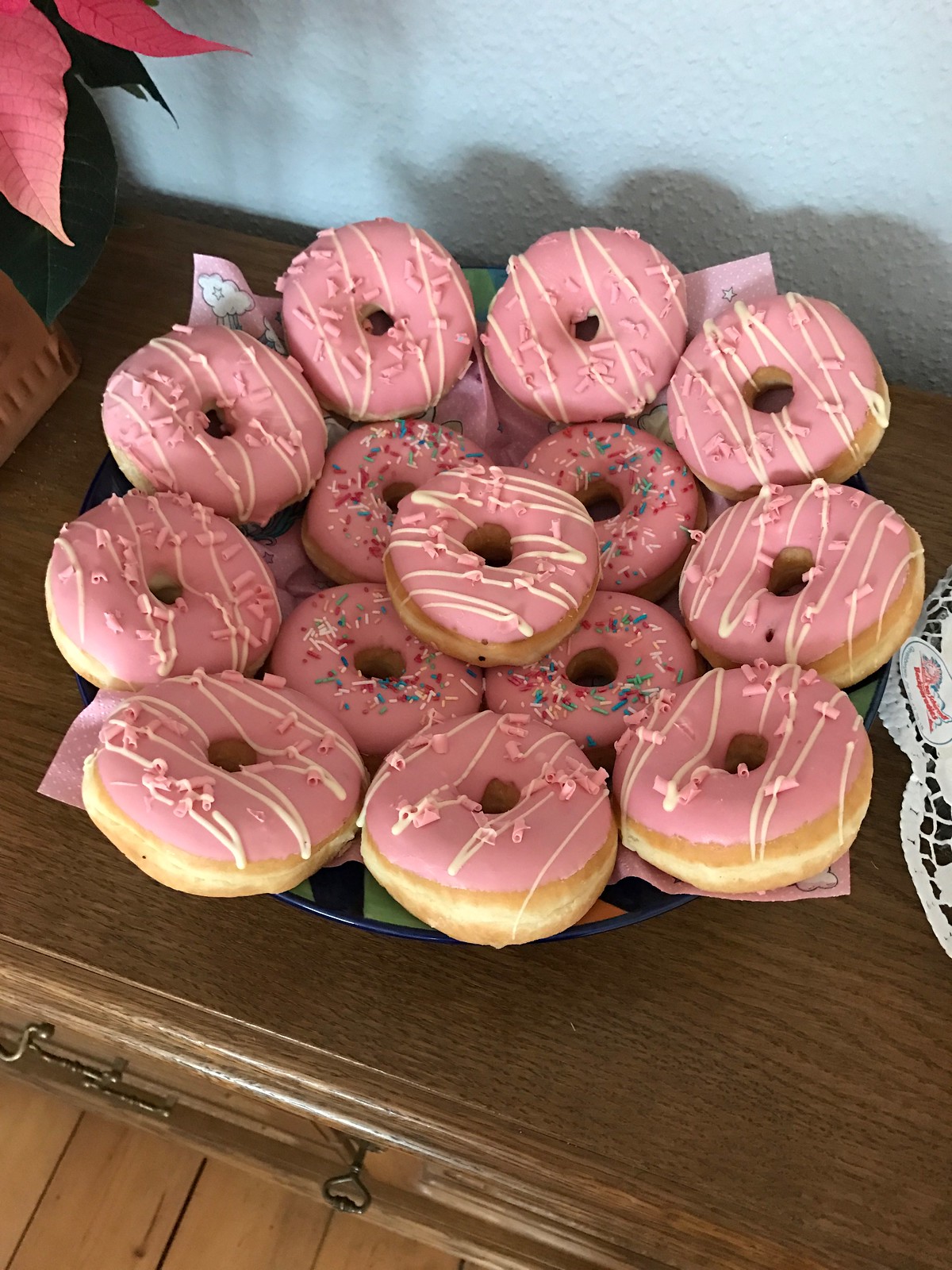This photograph showcases a large plate filled with 14 puffy donuts, prominently featuring bright pink frosting. Ten of the donuts are adorned with quick, back-and-forth stripes of white frosting, while the remaining four, positioned in the center, are garnished with multicolored candy sprinkles in blue, red, and white. The plate, sitting on a brown wood grain table, is lined with pink tissue paper decorated with little white clouds. To the right of the plate, a delicate laced doily peeks into view, suggesting the presence of another item just off-camera. In the upper left corner of the image, the vibrant tip of a poinsettia plant can be seen, adding a touch of greenery to the scene. The background features a white speckle finish wall, enhancing the warm, rustic atmosphere of the setting.